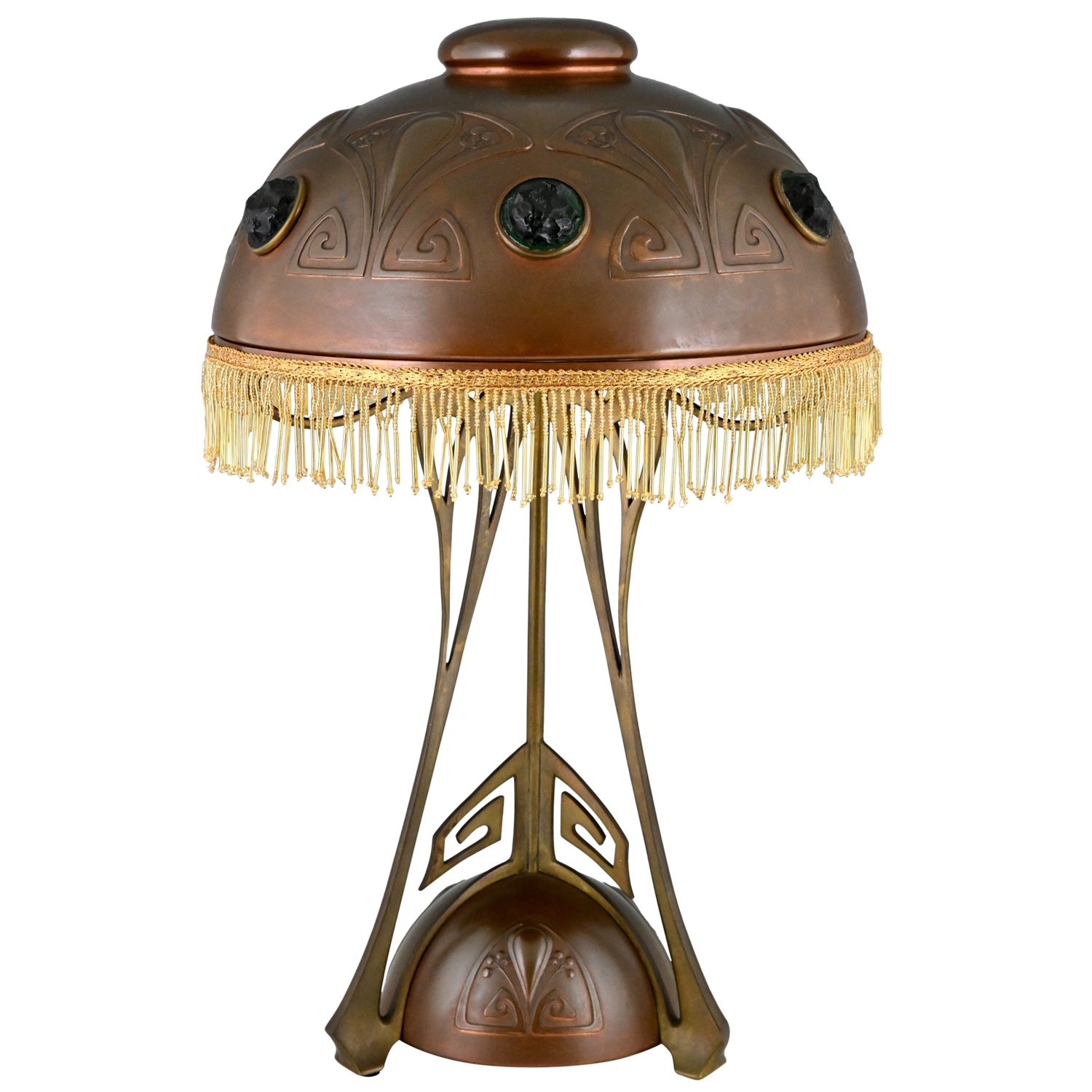The image depicts a vintage brass lamp with an intricate design, set against a completely white background. The lamp features an ornate metal structure with a top resembling an upside-down bowl, made of a brass material that has a swirly, textured pattern. The centerpiece of the top is adorned with three black-green gemstones bordered in gold. 

Descending from the metallic shade are short strings, reminiscent of curtain tassels, held together with lace. Two medium-length stands or pegs support the top, extending down to a similarly patterned bottom, also shaped like an upside-down bowl. The overall design employs a combination of copper and bronze elements, with additional golden accents, giving it a luxurious and intricate appearance.